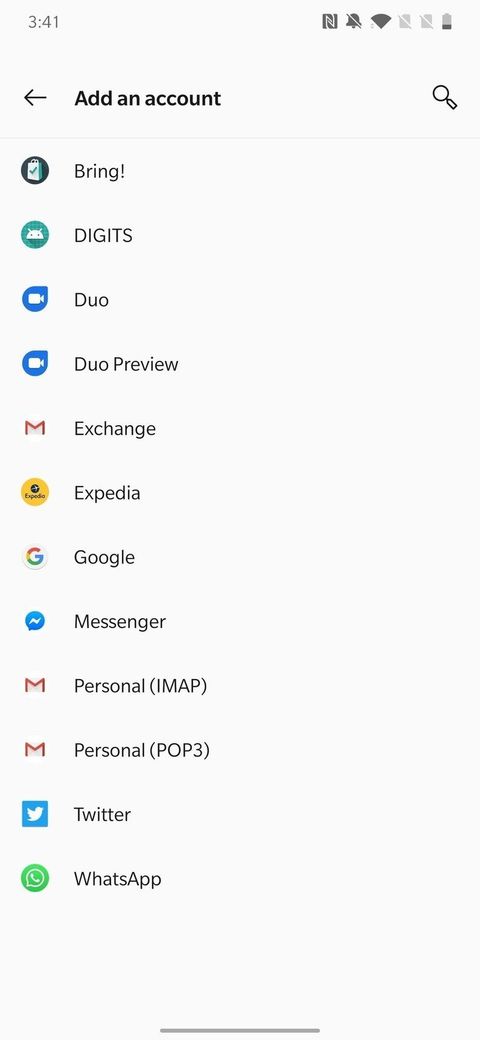This screenshot from an Android mobile app showcases the vertical arrangement of icons in a minimalistic display. The interface reflects a clean and organized layout typical of Android's design. In the top left corner, the time is displayed as 3:41. Adjacent to the right, several standard Android icons are visible, including the notification bell, Wi-Fi signal, and battery icon.

Beneath these status indicators, a prompt titled "Add an account" is flanked by a back button on the left and a magnifying glass (search icon) on the right. Following this, a list of applications and accounts is presented in a vertical sequence: Bring, Digits, Duo, Duo Preview, Exchange, Expedia, Google, Messenger, Gmail (Personal IMAP and Personal POP3 options), Twitter, and WhatsApp. It is important to note that the Gmail IMAP and POP3 options pertain to different email retrieval protocols.

The overall background color is a very light gray, bordering on off-white, which enhances the clarity and focus of the listed icons. At the bottom center of the screen, there is a subtle gray line, possibly serving as a visual delimiter or indicating a swipe-able section.